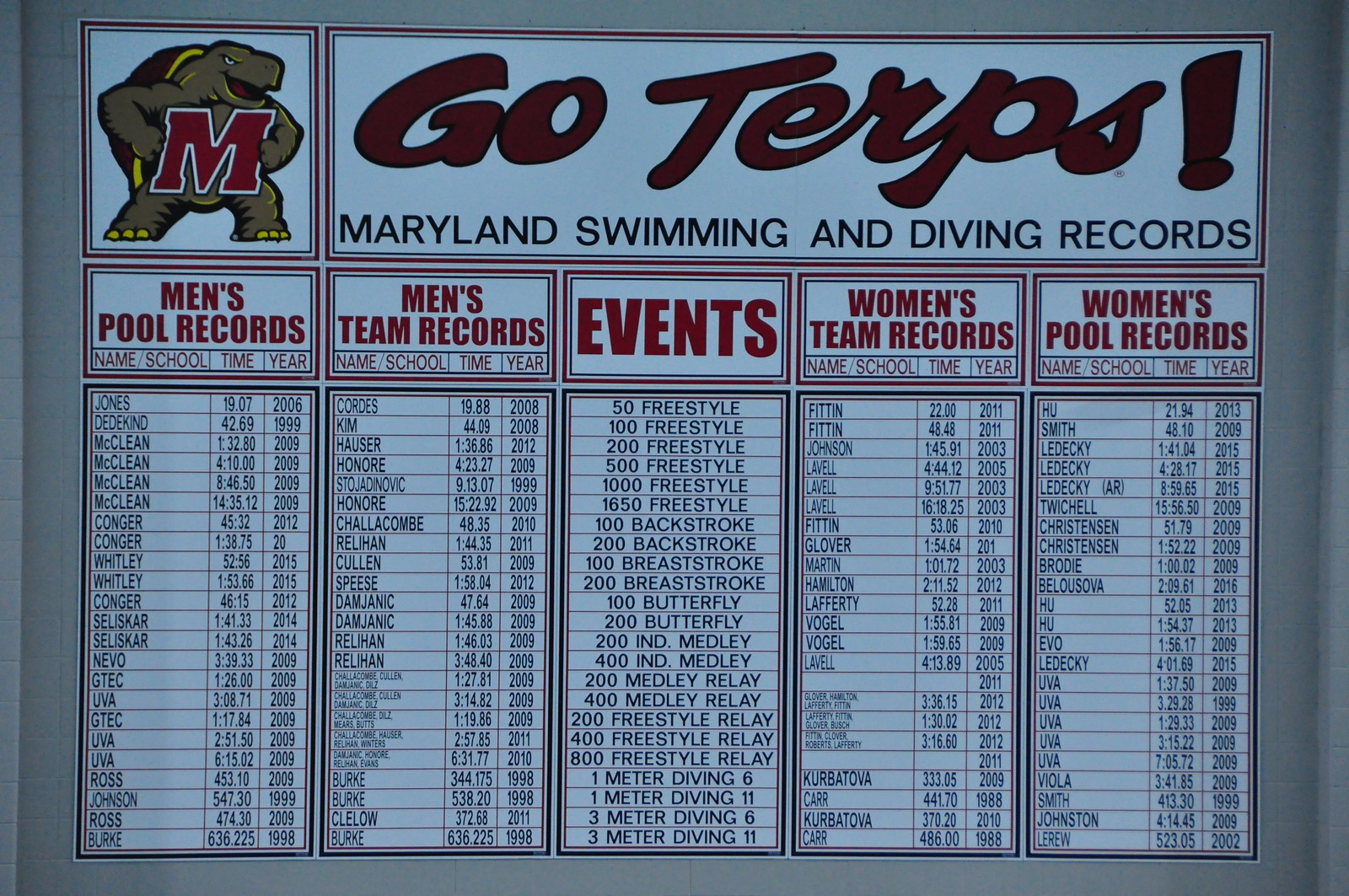The image showcases a detailed board of Maryland swimming and diving records. At the top left, there's a graphic of a turtle with a red shell and yellow lines, holding a large, bold red 'M'. To the right of this graphic, in prominent red letters, it says "Go Terps," with the word "Terps" stylized in cursive for the "ERPS" part. Beneath this, in black font, it reads "Maryland Swimming and Diving Records."

The records are organized into five columns. The first column is labeled "Men's Pool Records" and includes categories for name, school, time, and year. The second column, titled "Men's Team Records," also lists name, school, time, and year. The central column outlines various swimming and diving events in bold red font, such as the 50, 100, 200, 500, 1,000, and 1650 freestyle; the 100 and 200 backstroke; the 100 and 200 breaststroke; the 100 and 200 butterfly; the 200 and 400 individual medley; the 200, 400, and 800 freestyle relay; and the 1 meter and 3 meter diving events for both 6 and 11 dives.

The fourth column details "Women's Team Records" with similar subcategories of name, school, time, and year. The final column shows "Women's Pool Records," again divided into name, school, time, and year. The comprehensive layout presents a complete and structured overview of achievements in Maryland swimming and diving.